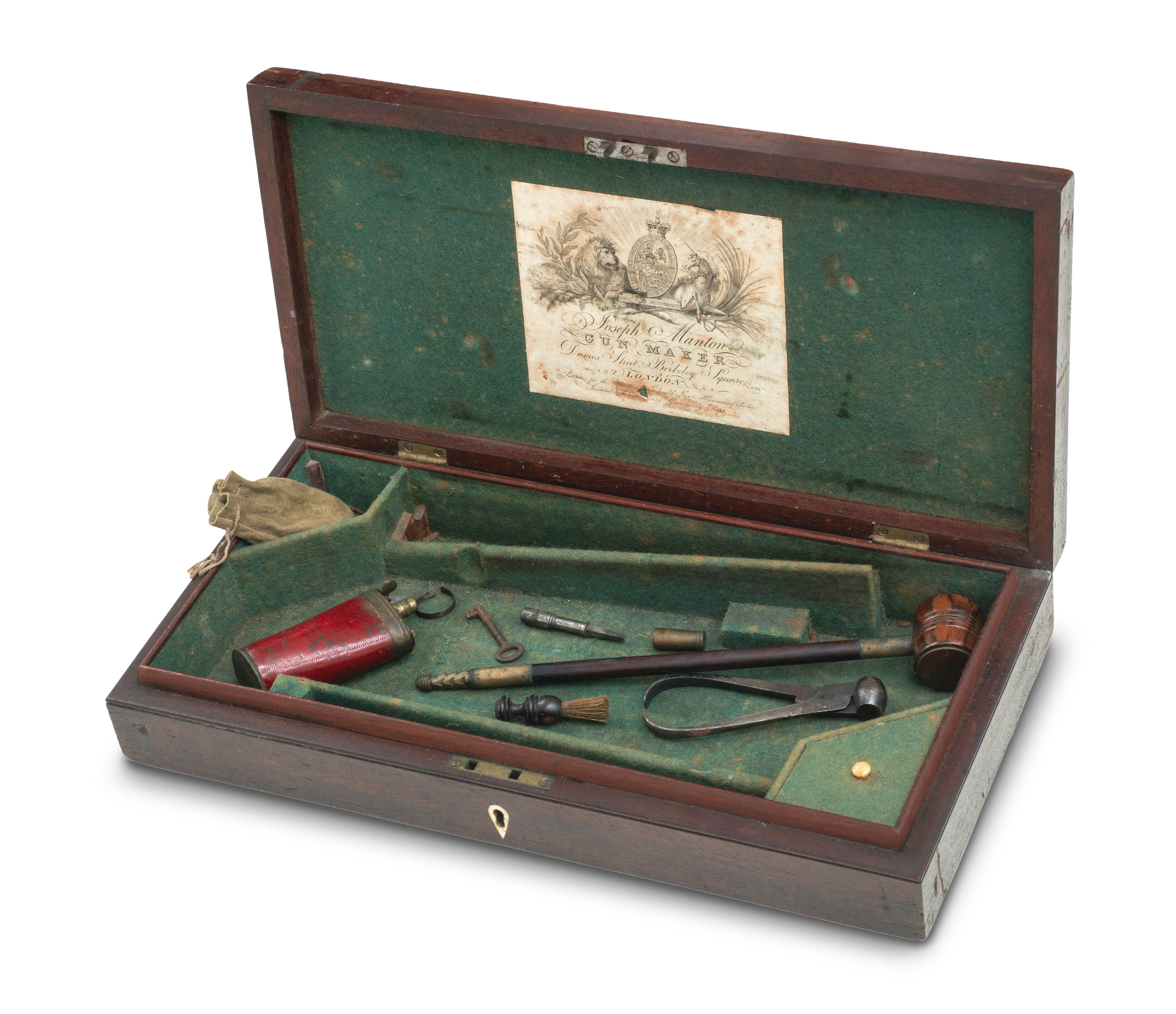The image depicts an old, brown wooden lockable box, which is quite worn and lined with green felt showing some splotches, possibly mold, indicating its age. Inside the lid, there is a white paper with an illustration of lions and the words "gun maker Joseph Manton." The interior of the box is segmented by raised felt sections, organizing various antique tools necessary for loading and cleaning a musket or black powder gun. Among the well-used contents, there is a red flask in the lower left section, a skeleton key, a small brush, pincers, light metal pieces, a powder measuring device, and a bullet-molding clamp that resembles a gavel. Although the toolbox contains only a few items, each seems purposefully designed for maintaining and operating historical firearms, capturing a bygone era with intricate, old-world craftsmanship.